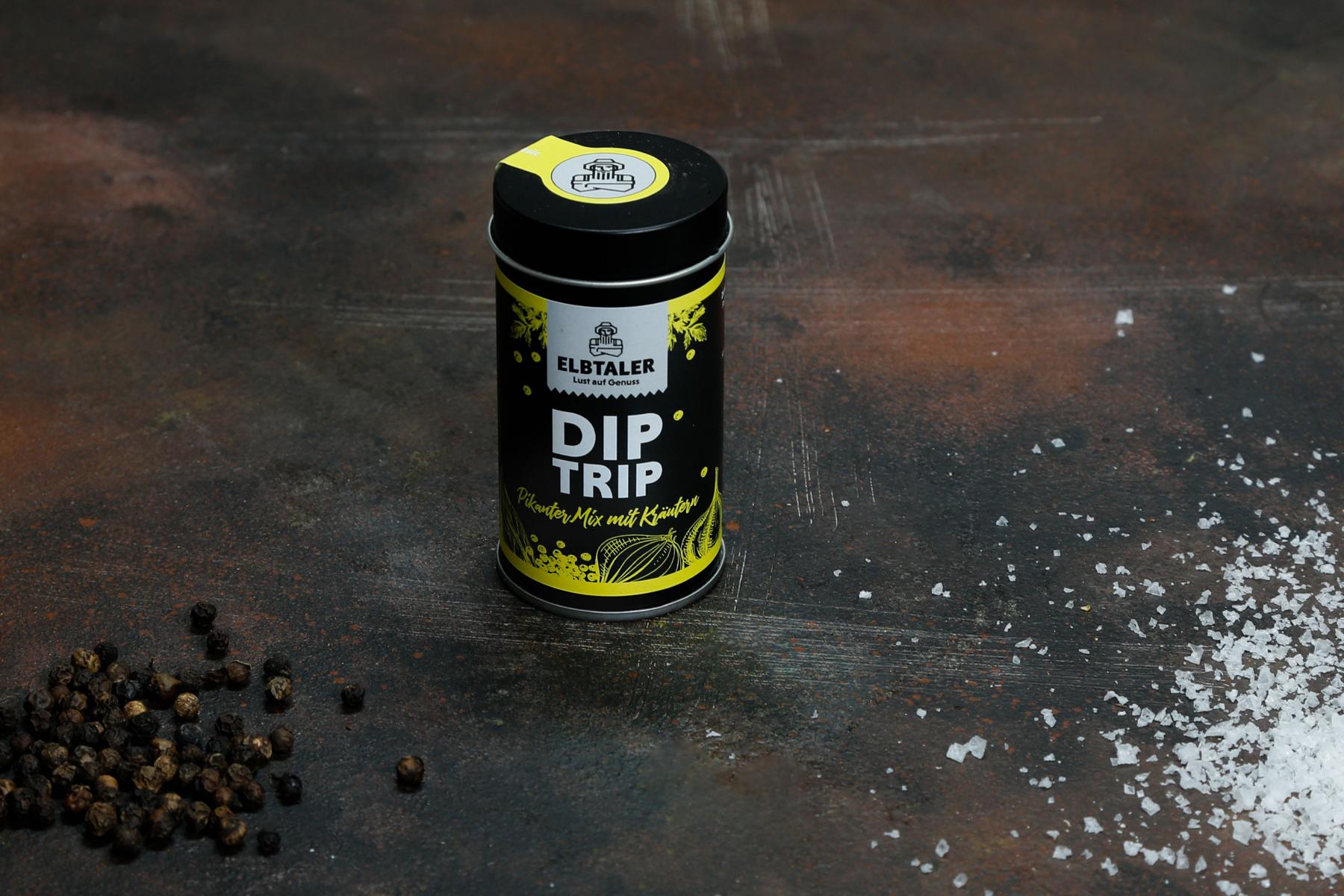In the image, there is a small cylindrical metal canister situated on a scratched and worn concrete floor. The canister itself is black with distinct yellow graphics and white lettering. In the center, the label prominently displays the words "diptrip" in white letters. Above this, another label reads "ELBTALER" with the same logo of a person with their hands folded, which is also featured on the yellow ring around the black cap. Below the word "diptrip," there are additional words in yellow letters, though they are not clearly readable, and it appears they might be in a different language. The top of the canister has a yellow label that seals it and extends down its side, featuring a white circle at the center that contains a black design.

Surrounding the canister, on the concrete floor, there are different scattered items. On the right side, there are fragments that resemble shattered glass or thick rock salts. Meanwhile, on the bottom left, there are small, dark brown and tan seeds that look like they could be peppercorns, nuts, bolts, or possibly cherry seeds, adding contrasting textures and colors to the scene.